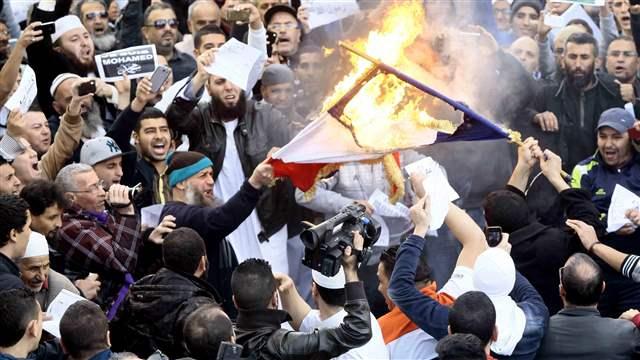In the image, a large crowd of men, predominantly of Arabic descent, are engaged in a protest that appears to be against the French depiction of Muhammad, likely rooted in the aftermath of the Charlie Hebdo incident. Central to the picture is a burning French flag, identifiable by the red, white, and blue colors that are barely visible through the flames. The protestors, some of whom are wearing traditional Muslim attire, including headdresses and various types of headgear like baseball caps and boggans, are fervently holding signs with "Muhammad" written on them. Additionally, there are people recording the event with cameras and cell phones, while others in the crowd look on, some actively participating by holding the flag as it burns. The scene is chaotic, with a mixture of brightly colored attire among the protestors, and the overall atmosphere conveys deep-seated anger and dissent.